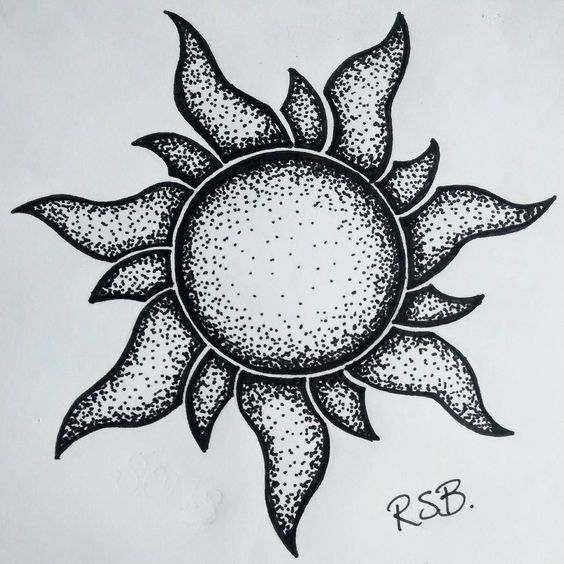This black and white illustration appears to be a tattoo design, featuring a stylized sun. The sun itself is a textured circle, intricately dotted to resemble the surface of an orange. Surrounding the sun are thick, curly flames, some long and some short, creating a dynamic, kinetic effect. The alternating lengths of the flames add to the overall sense of movement and intensity. The artwork exudes a 90s aesthetic, reminiscent of album covers from that era, such as those by the band Sublime. The initials "RSB" suggest the artist's identity.